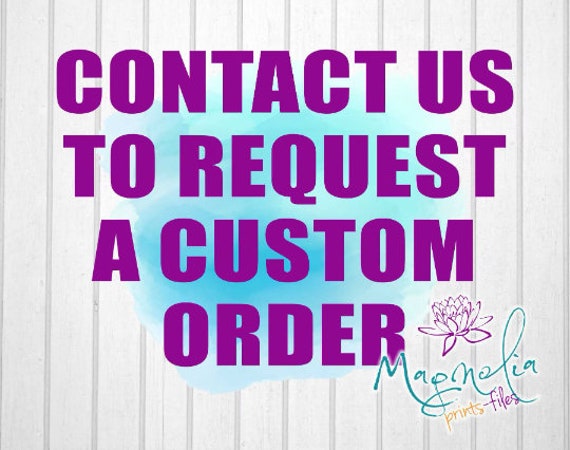The image is an advertisement with a white-panel background featuring narrow gray vertical lines. The foreground is dominated by bold, violet-purple letters reading "Contact us to request a custom order", set against a light blue, cloud-like splash to highlight the text. In the bottom right corner, there's a sketch of a lotus-style flower in purple. Below the flower, the name of the business is displayed: "Magnolia Prince Files." "Magnolia" is written in a teal color, "Prince" is in yellow, and "Files" is in purple.